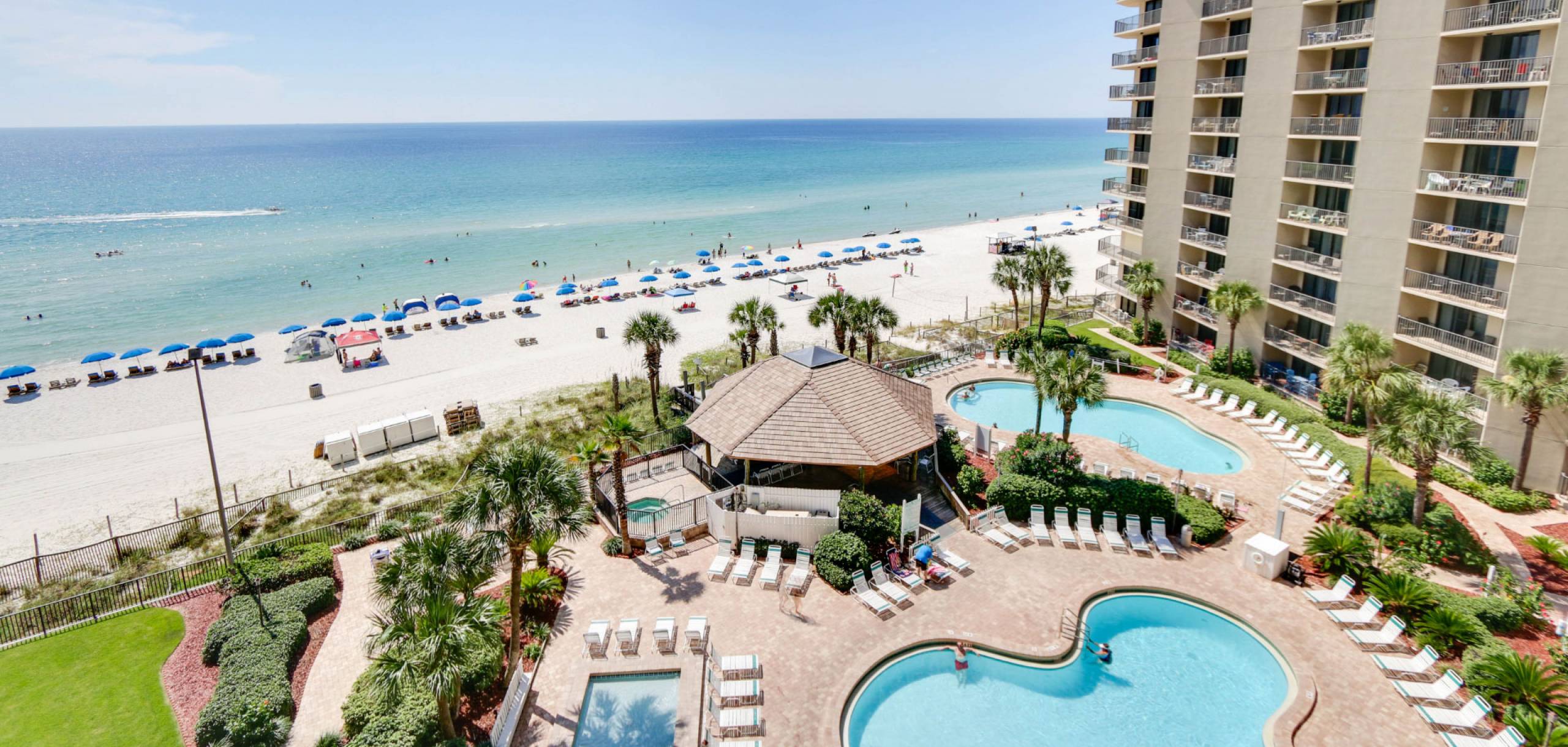This photorealistic aerial image captures a vibrant, tropical beach resort on a bright, sunny day. In the foreground, a set of clear blue pools with curved shapes, reminiscent of Mickey Mouse ears, are lined by white deck chairs and surrounded by lush green palm trees. A gazebo for lounging is situated towards the middle back, near the pools. Scattered across the patio area are several guests relaxing on deck chairs, with four people enjoying the refreshing pools—two in the primary pool and two in a smaller pool further away. To the right, a brown hotel with balconies adorned with various furniture and clothes rises up, providing a picturesque boundary to the pool area. Beyond the pools, a pristine, calm beach appears, adorned with innumerable blue umbrellas and chairs along the shore. People can be seen enjoying the ocean, where a boat or jet ski adds to the lively atmosphere. The clear blue sky enhances the inviting appeal of this idyllic resort setting.